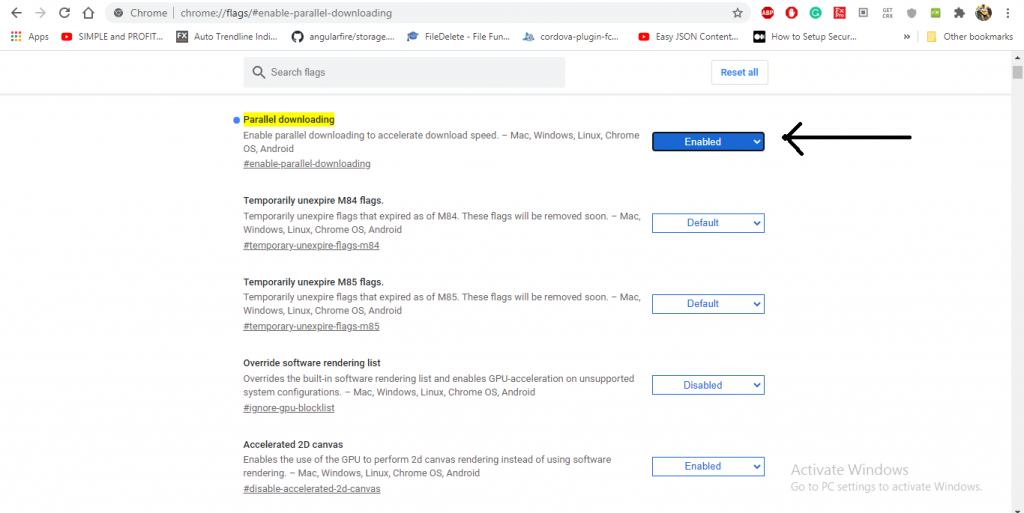Screenshot Description: 

The image appears to be a screenshot of a Google Chrome web browser window, displaying the internal settings page dedicated to configuring flags for advanced features. Specifically, it shows the "chrome://flags/#enable-parallel-downloading" page.

At the very top of the screenshot, the Chrome browser interface is visible with the standard icons: home, back, reload, and the address bar which reads "chrome://flags/#enable-parallel-downloading." To the right of the address bar, several extension icons are visible, including one for DuckDuckGo.

Below the address bar, a bookmarks bar is present, featuring partial names of bookmarks such as "Simple and Profit" and "Audio Trending."

The main content area displays the settings for "Parallel Downloading," with a search bar at the top of the page labeled "Search flags," and a "Reset all" button to its right in blue text on a white background. The first setting, “Parallel downloading,” is highlighted in yellow. To the left of this, a blue circle is visible, signifying the option to enable it. The description underneath reads: "Enable parallel downloading to accelerate download speed. Mac, Windows, Linux, Chrome OS, Android." The word “enable” appears as a link at the bottom of the description.

To the right of this, a blue "Enable" button is available next to a drop-down menu, and a black marker-drawn arrow points to this button. 

Additional flag options listed below include:
- Temporarily only expire M84 flags (default),
- Temporarily un-expire M85 flags (default),
- Override software rendering list (disabled),
- Accelerated 2D canvas (enabled).

At the bottom right corner of the screenshot, there's a watermark that reads: "Activate Windows, go to PC settings to activate Windows," suggesting that the screenshot was taken on a non-activated copy of Windows.

Overall, the screenshot captures a detailed view of changing advanced settings in Chrome to improve download speeds, while also noting that the system is running an unactivated version of Windows.